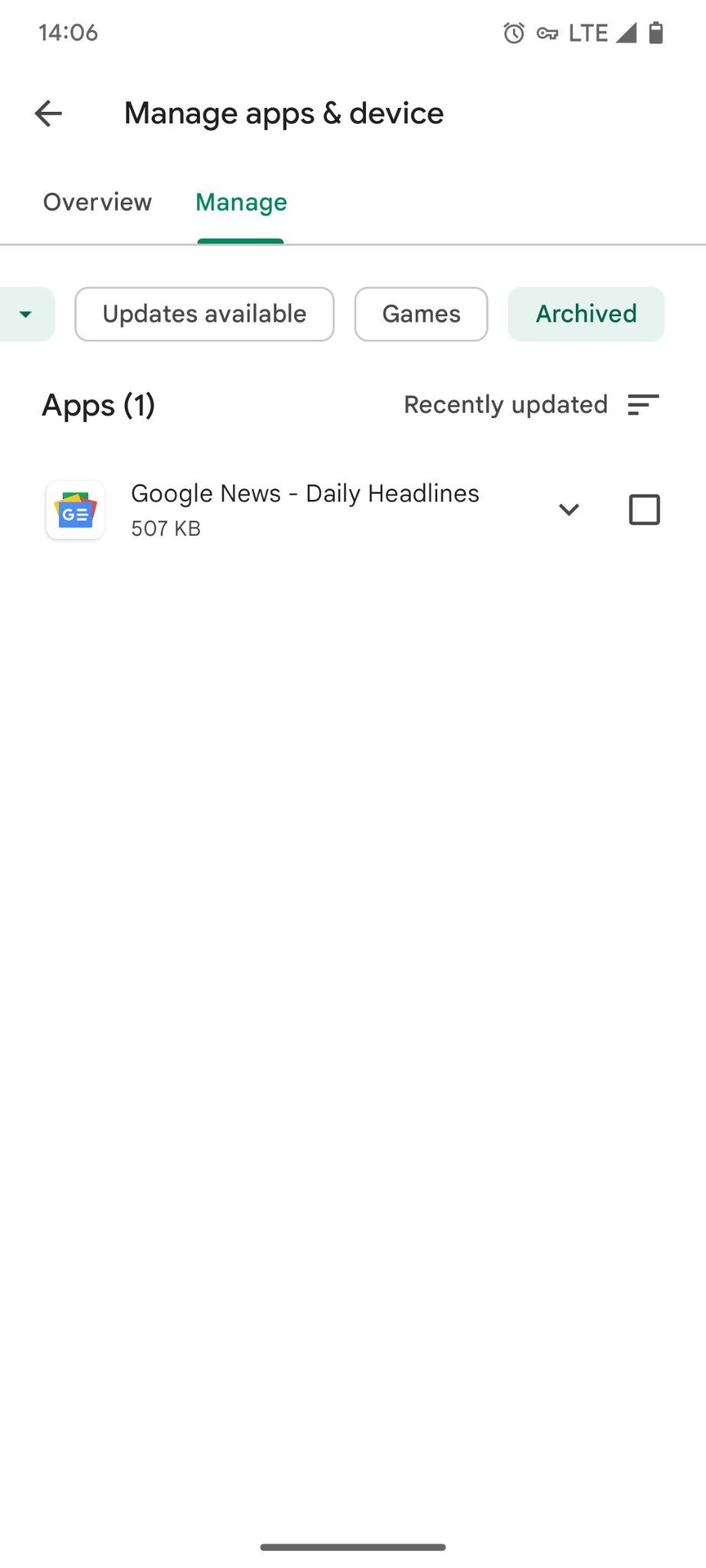The image depicts the settings screen of a smartphone. In the upper right-hand corner, the LTE signal bar, battery life indicator, and an alarm clock icon are visible. Within the settings, the user is currently in the "Manage Apps & Device" section. This can be discerned as the "Managing" tab is highlighted in a light blue-green color, while the "Overview" tab is gray and unselected.

In the "Manage" section, options such as "Updates available," "Games," and "Archived" are presented, with "Archived" currently being selected, as indicated by its light blue-green highlight. The other two options, "Games" and "Updates available," remain gray and unselected. The screen shows that one app, Google News, is archived. The user has clicked on Google News, as evidenced by the app's details being displayed, but no further actions (such as managing or deleting the app) are currently selected. The user appears to be considering their options regarding the archived Google News app.